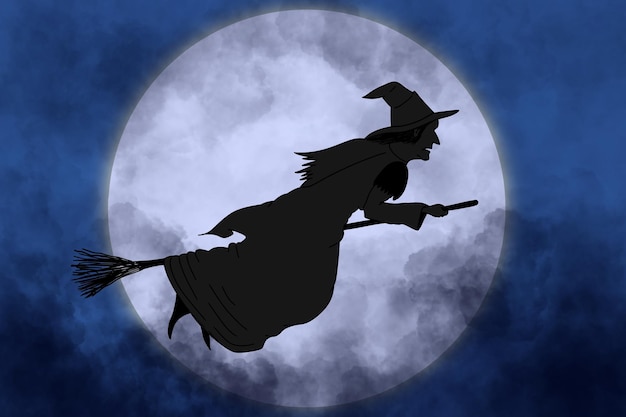The illustration depicts a classic witch in vivid detail, rendered in black relief against a massive, silvery moon that dominates the center of a landscape-oriented image. The night sky surrounding the moon is a complex tapestry of deep blues and purples, accented by translucent, shadowy clouds. The witch, dressed in a long, flowing black dress, is unmistakably witch-like, with a pointed hat, long black hair, a pronounced nose, and a prominent chin. Her right hand grasps the broomstick while her legs and feet dangle below. The broomstick itself, adorned with a bunch of unruly twigs at the end, stretches from the center of the moon to the left side of the image. The witch’s mouth is slightly open, giving the impression of movement as she flies to her right.